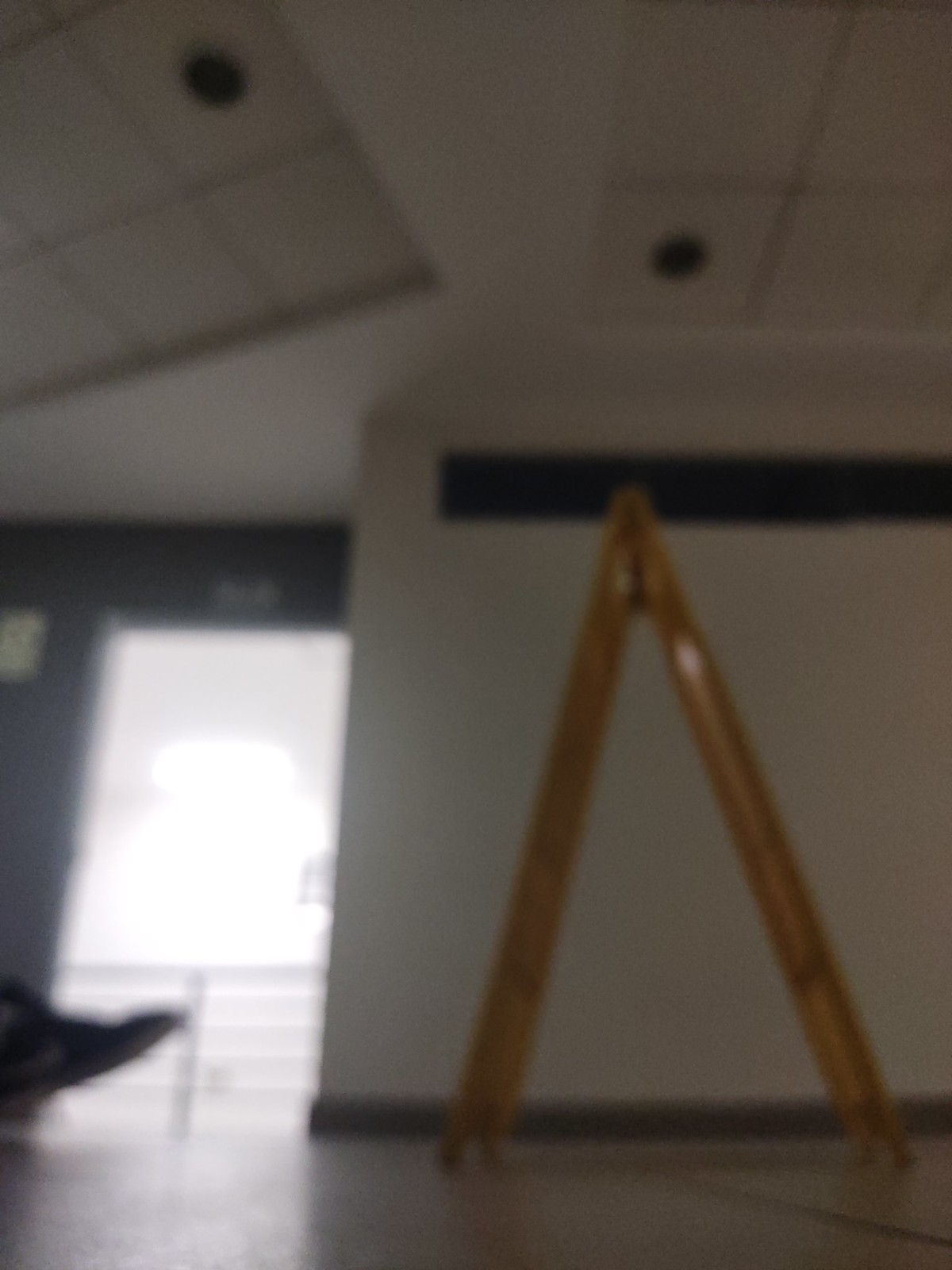The image depicts a blurry and dimly lit indoor scene that appears to be taken in a mall, office, or possibly a school hallway. Prominently on the right-hand side of the photograph is a freestanding A-frame ladder, colored orange or yellow, positioned next to a white wall that features a large gray stripe along its upper portion. The wall rises only halfway up the frame and then opens onto a landing or hallway area with an open railing and a window or door that allows some sunlight to filter through, which is the primary light source in the image. The gray or dark gray wall framing this opening creates a noticeable contrast with the white wall. Farther in the background, there appear to be ceiling tiles, some with circular cutouts presumably for fixtures like speakers, smoke detectors, or fire alarms. Near the middle to the left of the image, there’s a partial view of an individual’s foot, angled as if mid-step, adding a sense of movement to the scene. Additionally, there is an unidentifiable dark shape near the background, which is indistinct due to the low resolution and overall blurriness of the image.